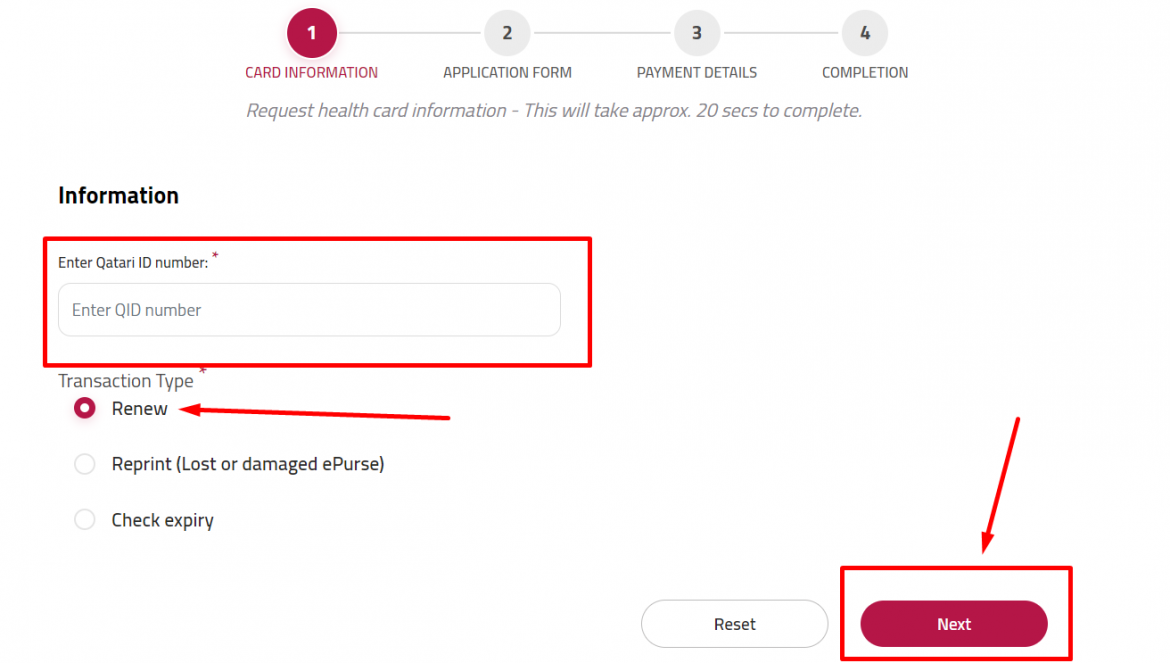The horizontally rectangular image depicts a screenshot from an online tutorial demonstrating a multi-step process. The interface shows four steps, with "Card Information" being the current step, highlighted in burgundy, while the other steps - "Application Form," "Payment Details," and "Completion" - are in gray. Below the step indicators, a title reads "Request Health Card Information" with a note stating that this process will take approximately 20 seconds to complete.

On the left side, a bold black heading labeled "Information" appears, followed by a section framed in a red border. This section prompts the user to "Enter Qatari ID number" within a specified field. Below, users can choose the type of transaction from a list with circular buttons: "Renew," "Reprint," "Lost or Damaged E-Purse", and "Check Expiry." The "Renew" option is currently selected, emphasized by a red arrow pointing at it from right to left.

At the bottom right of the frame, two buttons are displayed: "Reset" and "Next." The "Next" button is also outlined in a red border with a red arrow pointing from top to bottom, guiding users towards proceeding to the next step.